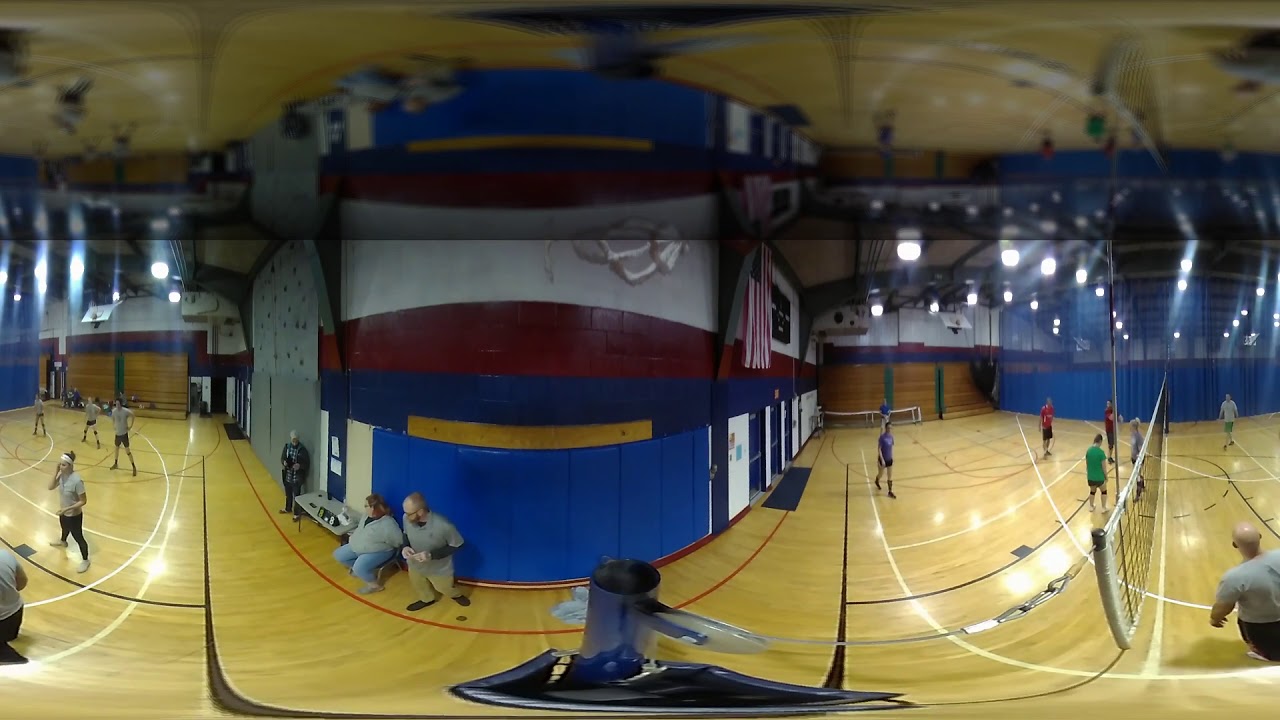This detailed photograph captures the energetic atmosphere of a school gymnasium during an active volleyball game. Shot with a 360-degree perspective, the image is highly distorted, giving a cylindrical effect as if the left and right sides touch in the back to create a continuous scene. On the far left, players in gray shirts, one partially visible in the lower left corner, are preparing or resting. As we move to the center, three spectators sit at a table, observing the game with intent. They are framed by the gymnasium's walls, which are predominantly blue with padded sections, a red upper part with gray details, and a rock climbing wall surrounded by protective pads. The game unfolds beneath a net strung across the floor, extending into both sides of the image. On the far right, completing the full circle, are players in vibrant red, green, and purple shirts, the other half of the athlete seen on the left now emerging from the lower right corner. The standard brown gymnasium floor and minimal audience complete the scene, with a unique horizontal line two-thirds up, adding a mirrored ceiling effect that captures the bustling essence of a school sports event.